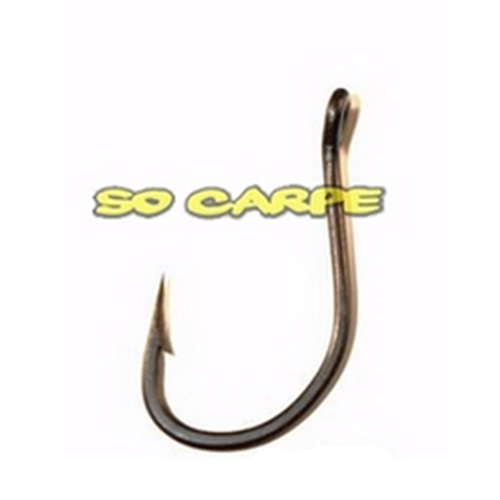The image depicts a large, shiny silver fishing hook against a pure white background. The hook is oriented with the point on the left, curving upward to the right, where there is a round hole designed to attach it to a fishing line. A distinctly sharp barb is positioned just below the curve of the hook. The hook is quite wide and substantial in appearance, differing from the more classic, narrower designs. Overlaid on the image is bold, graffiti-like text that reads "SO CARPE" in yellow, all capital letters. The font is thick, urban in style, and outlined in black, making the text stand out prominently against the white background.